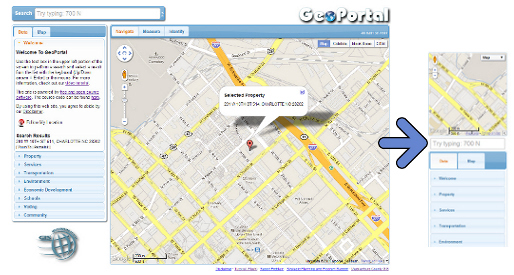In this image, the text appears blurry, but visible elements provide significant context about its content. At the top left, there's a search bar with a blue background, while the text input area has a white background. The text inside the search bar prompts, "Try typing 700 N." The top right corner displays the word "GeoPortal" in white, with the 'O' stylized as a world map or globe. 

The left-hand side of the image greets the user with "Welcome to GeoPortal," although the smaller black text below is illegible. At the bottom of the screen, there are several tabs such as "Property," "Services," and "Community," written in blue text.

The central section features a detailed map. This map displays yellow and orange roads, indicating different types of routes, with a prominent orange main road. A red location pin is positioned on the map, accompanied by small, white, unreadable text. On the far right, a blue arrow points to the right, suggesting navigational aid.

Additionally, the user interface of the GeoPortal appears consistently across devices. The central view, likely from a computer, matches the layout on the smartphone displayed on the right. Both interfaces showcase the same search bar prompt, tabs, and map, ensuring a uniform user experience regardless of the device used.